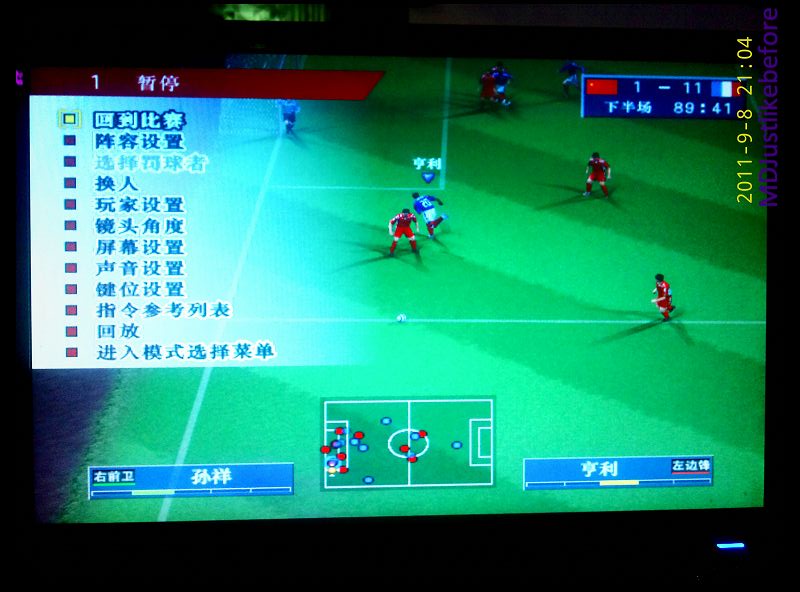The image is a detailed screen capture from a computer game depicting an animated soccer match between two teams. The game shows a green soccer field with light green marking lines. One team is dressed in red jerseys, while the other wears blue jerseys with white pants. The red team is arranged in a triangular formation with three players shown, while two players from the blue team are visible. On the left-hand side of the screen, inside a rectangular area, there is writing in an Asian script, possibly Chinese, Korean, or Japanese characters, indicating scores or team information. In the bottom middle of the screen, there is a mini-map of the soccer field displaying player positions. The bottom left corner has a blue strip, possibly a time indicator, and the bottom right contains another blue slider. On the top right, a timed date stamp reads "2011-9-8" at "21:04" in yellow font. Additionally, a blue rectangular box in the upper right corner displays the flags of China and France, indicating the competing teams. The score shows that the French team is leading 11-1, with the game time at 89:41.